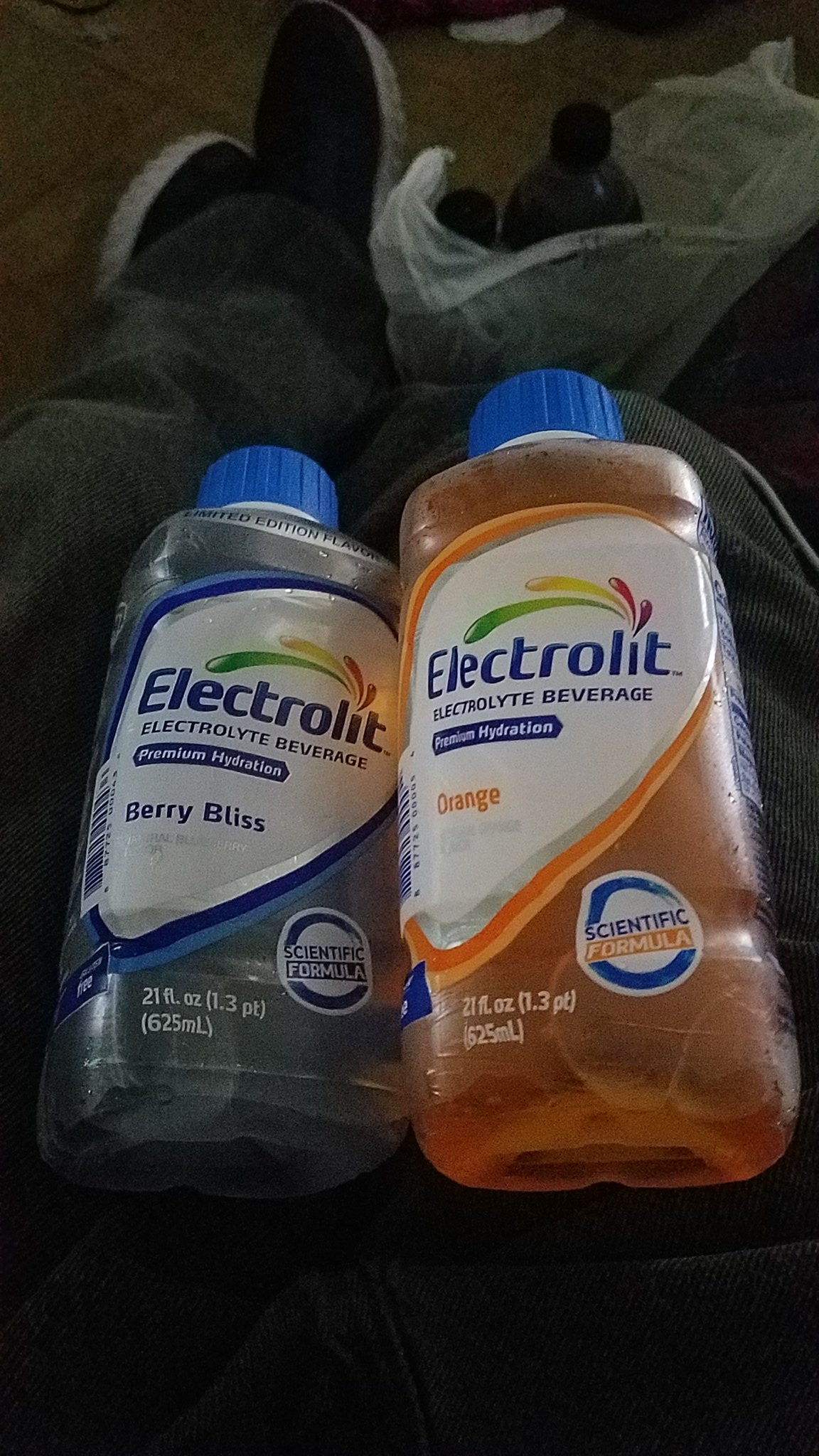In a dimly lit room, a photograph captures a moment of stillness as an individual, dressed in dark green pants, photographs two electrolyte drink bottles resting on their lap. Their outstretched legs, adorned in black shoes with gray soles, extend to the edge of the frame. The bottles, encased in a white, partially transparent bag, appear vibrant and eye-catching. The left bottle, labeled "Berry Bliss," is filled with a blue-green liquid, while the right bottle, marked "Orange," holds a bright orange fluid. Both bottles, with their black caps and clear branding "Electrolyte Beverage Premium Hydration," also display a smaller logo indicating "Scientific Formula, 21 fluid ounces, 1.3 pints, 625 milliliters." The careful positioning of the bottles on the individual's lap, framed by the subdued lighting of the room, creates a visually intriguing composition, emphasizing the contrast in colors and showcasing the details of the electrolyte drinks.